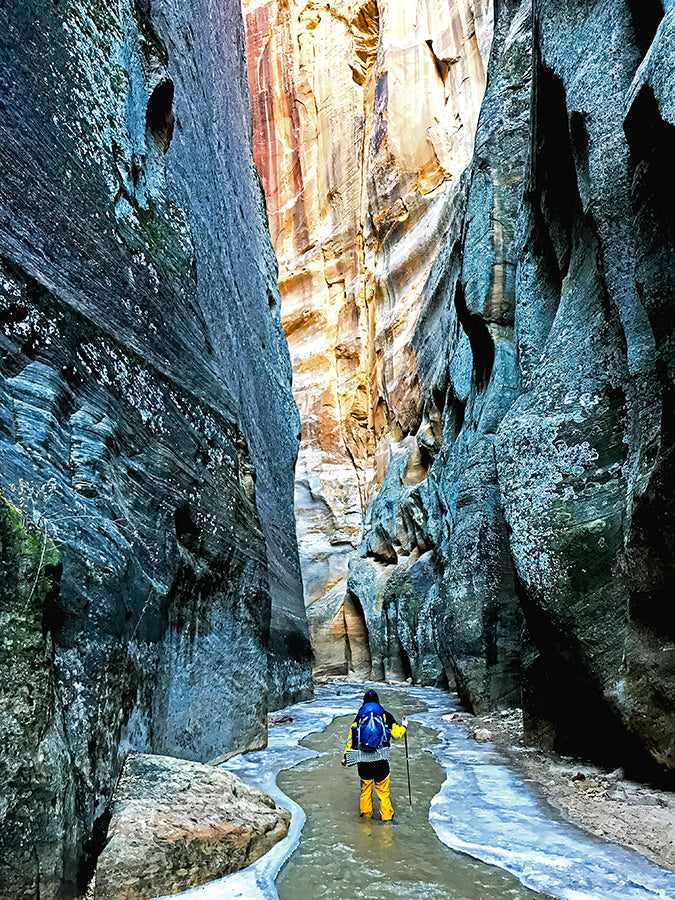In the photograph, a man is wading through a shallow creek bed flanked by towering rock walls on both sides. The man, facing away from the camera, is clad in yellow rain slicker waders paired with black shorts, and sports a matching jacket. His right arm is extended forward, gripping a walking stick or trekking pole. Strapped to his back is a dark blue backpack with a gray bedroll attached at the bottom.

The creek water, clear enough to reveal the tan sand beneath, comes up to his ankles and has white foam lining the edges. The rock walls enclosing the creek on the left and right are mottled with shades of gray, steel gray, and dark green, speckled with white flecks. As the creek bed stretches into the distance, it dead-ends at a very tall, steep, and flat rock wall that exhibits a tan and creamy hue with white tones near the base.

The gorge is illuminated by daytime light, though the sun is not visible. Some sections of the rock formation near the platform on the left show a distinct orange color. The scene is serene yet rugged, capturing the essence of a peaceful hike in a striking natural landscape.